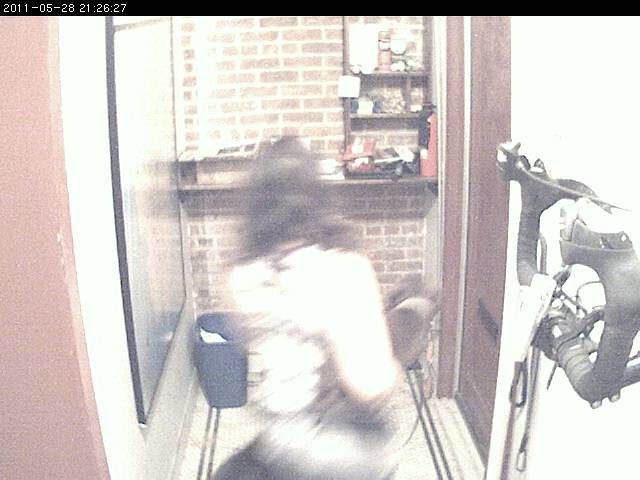The image captures a somewhat distorted scene due to a shaky camera perspective. The photograph features a woman with long brunette hair, viewed from behind, making her facial features indistinguishable. She is donned in a long-sleeved shirt and appears to be sitting on the floor. To her left, there is a mirror, while to her right, a piece of gym equipment is vaguely visible, suggesting it might be an exercise machine.

The setting is a very small room, possibly a closet or an enclosed foyer. On the right side of the image, a door with a mail slot, indicative of a front entrance, is present. The woman faces a brick wall adorned with a shelf filled with various objects. A small black wastebasket is also positioned near her. The confined and cluttered space, coupled with the presence of both domestic and fitness-related items, adds an element of intrigue to the scene.